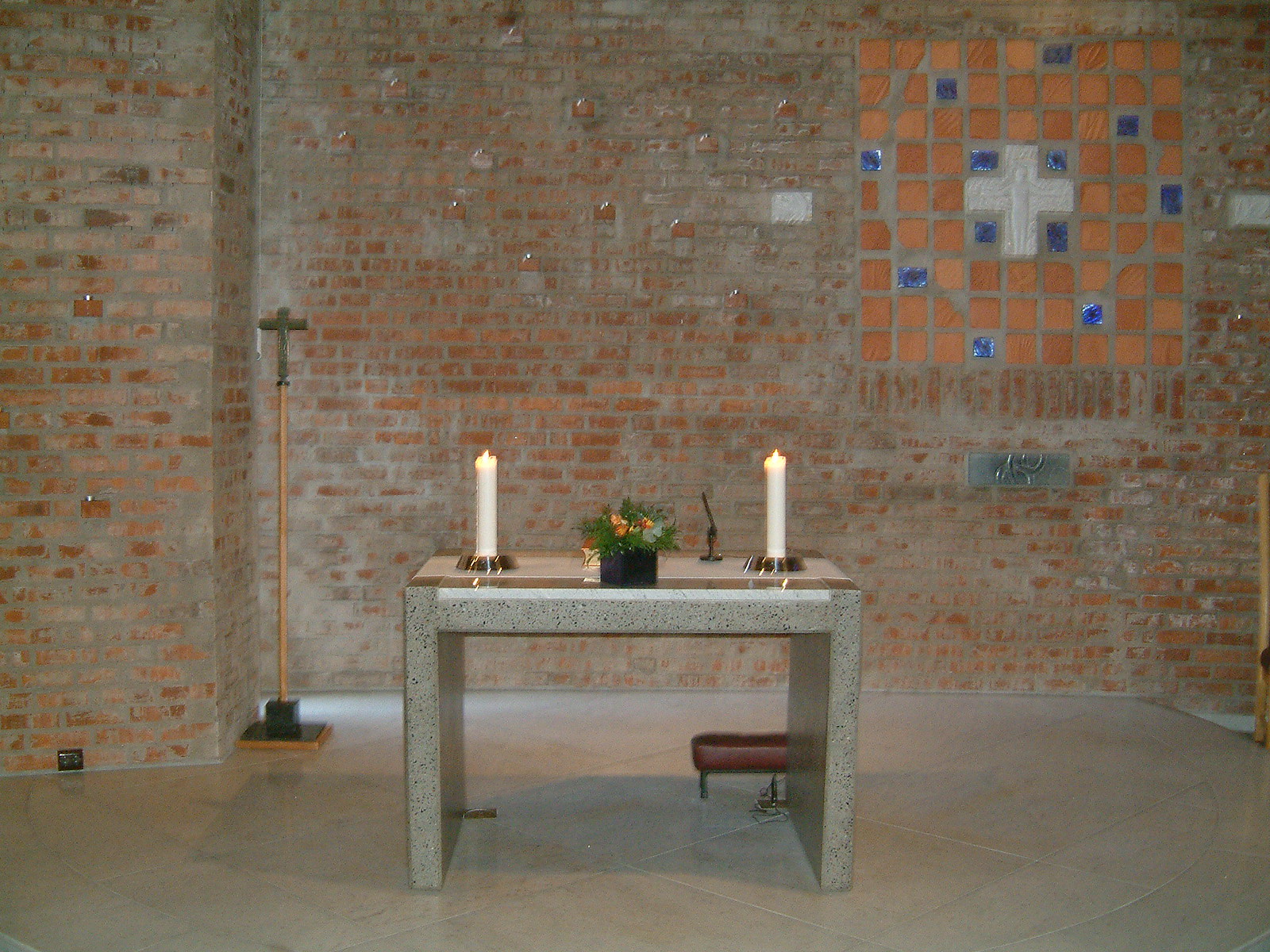This image depicts an indoor setting within what seems to be a religious building, characterized by a prominent brick wall. The room's focal point is a centrally positioned square altar table adorned with a gold rim around its base. On the altar, there are two tall, lit white candles positioned on either side, and a potted plant in the middle, likely artificial. Beneath the altar, there appears to be a kneeling bench. The floor is tiled in gray, adding to the room's sparse and solemn atmosphere. The left corner features a standing cross. Additionally, the upper right section of the brick wall showcases a window or a pattern resembling stained glass, containing squares of blue and orange and a white cross in the center. There are also chairs positioned at the bottom of the image. The room is illuminated with natural light, suggesting it is taken during the day. No text is visible in the scene. The color palette includes variations of white, off-white, yellow, gray, brown, orange, and blue.